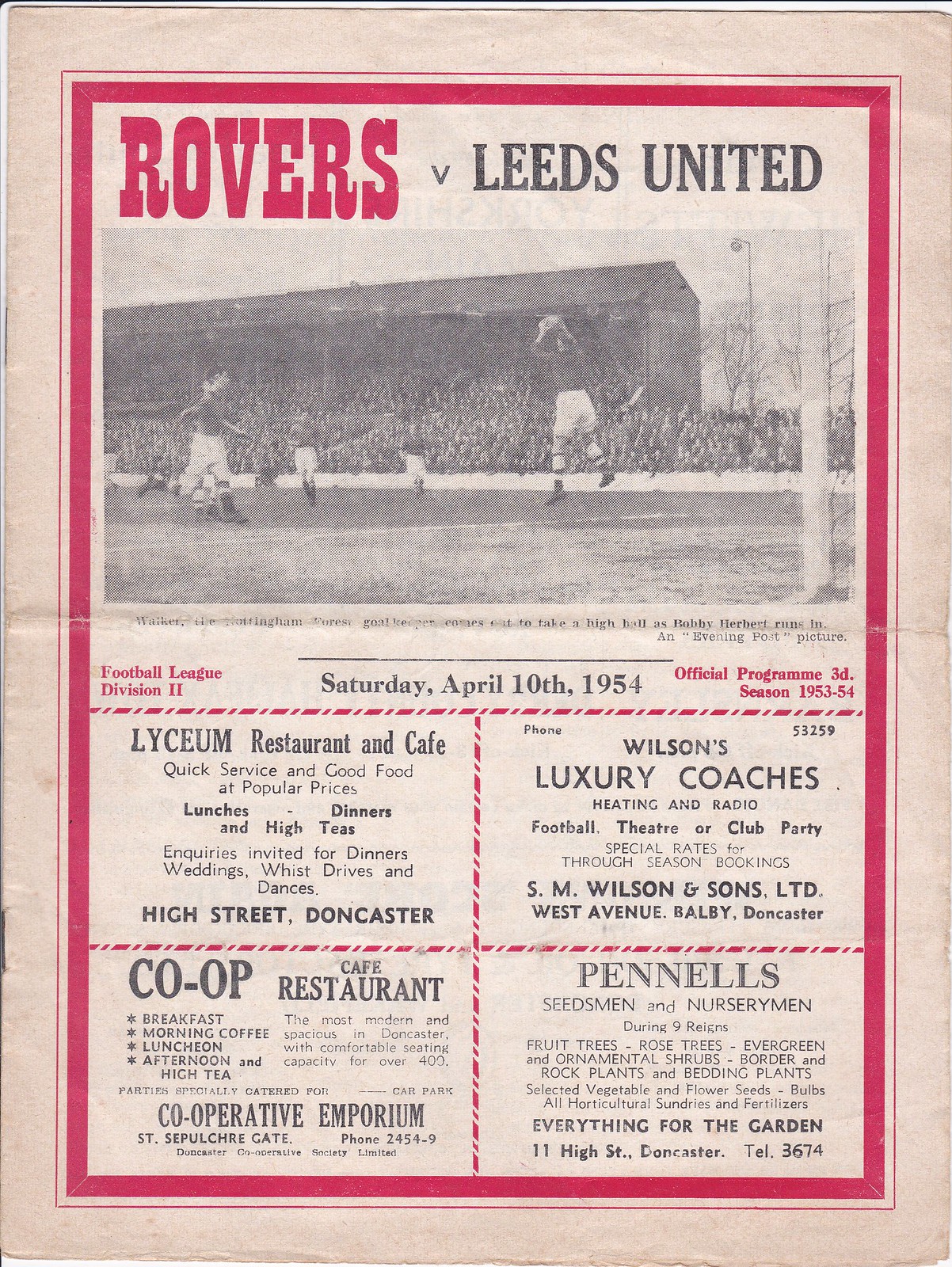This image is of an ancient-style rectangular poster promoting a soccer match between the Rovers and Leeds United. The poster features a distinctive pink border with a lighter pink outer edge. At the top of the poster, the heading "Rovers vs Leeds United" prominently appears, with "Rovers" in pink and "Leeds United" in black. Directly beneath this heading is a black and white photo depicting players in action on a football field. The text underneath the photo reads "Saturday, April 10th, 1954," indicating the date of the match. Towards the bottom of the poster are four rectangular sections containing advertisements for local businesses, including Lyceum Restaurant & Cafe, Wilson's Luxury Coaches, Co-op Cafe Restaurant, and Pinnell's. Each advertisement features a paragraph of text describing the services offered. The overall appearance of the poster is somewhat faded, enhancing its vintage charm.